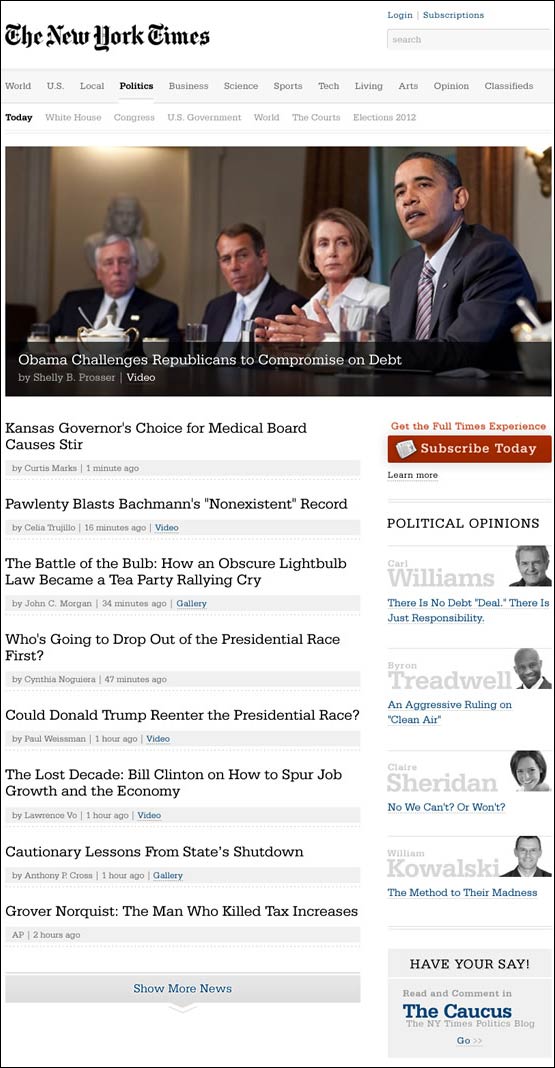This is a detailed description of the New York Times website's front page. The background is predominantly white, and at the top left corner prominently features the iconic New York Times logo. Dominating the top section of the webpage is a large, eye-catching photograph, overlaid at the bottom with a semi-transparent black bar. On this bar, to the left, there is an eye-grabbing headline that reads, "Obama Challenges Republicans to Compromise on Debt." Beneath this headline, the author's name is displayed on the left, while to the right, the word "Video" appears in small white letters, indicating multimedia content.

Running vertically down the left side of the webpage is an extensive list of article titles, all presented in bold. Each entry includes additional details such as the posting time, view count, and the author's name. Adjacent to this list, on the right side of the page, is a red bar marked with a call to action reading "Subscribe Today." Further down, towards the center right section, there is a dedicated area for political commentary, titled "Political Opinions" in bold. This section features four thumbnail images of various contributors, with their names positioned to the left of each thumbnail image.

At the very bottom of the webpage, there is an interactive section inviting reader engagement, labeled "Have Your Say." This is followed by a section titled "The Caucus," highlighted in blue letters, indicating a forum for public opinion and discussion.